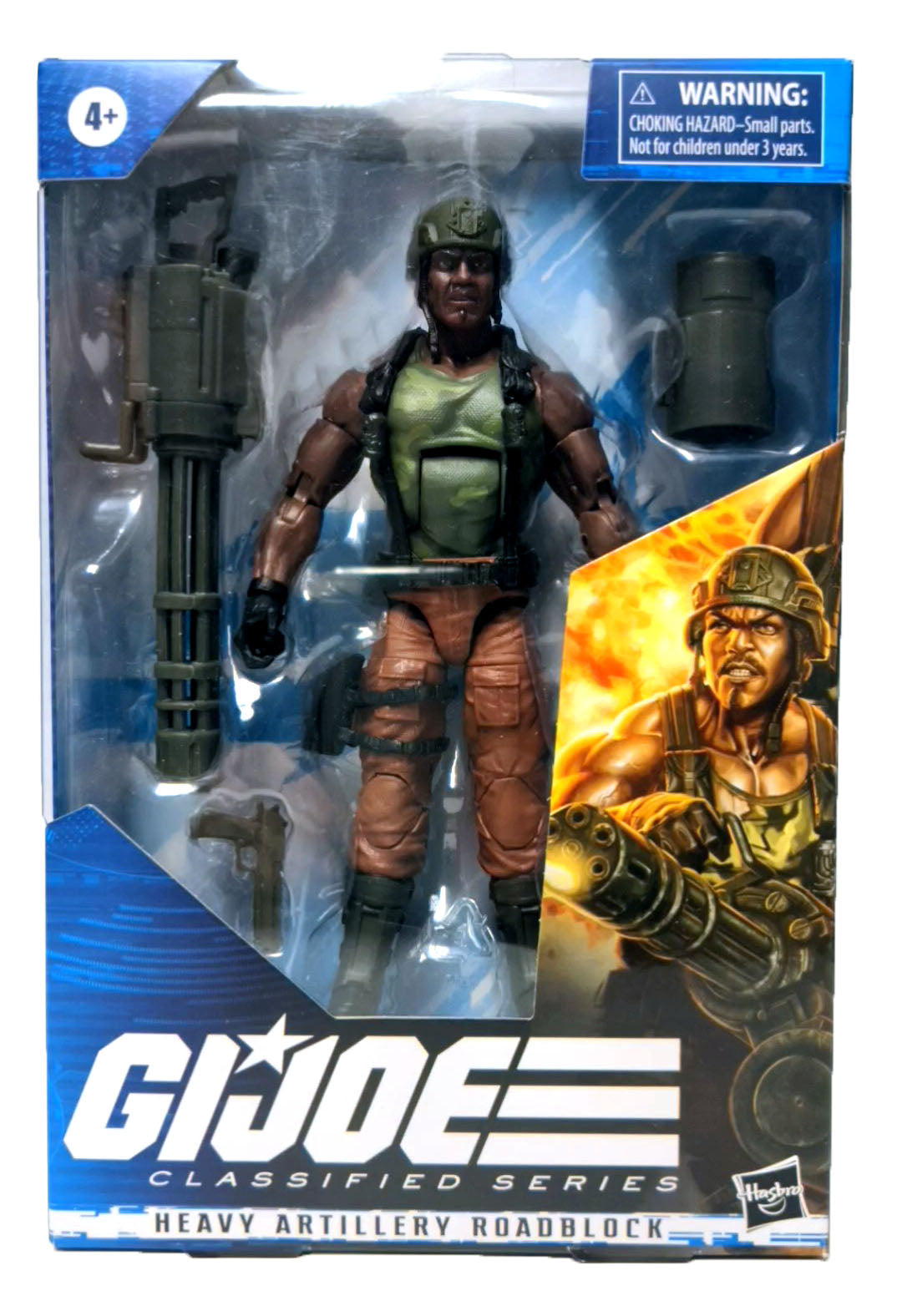This rectangular color photograph showcases a G.I. Joe action figure named "Heavy Artillery Roadblock" in its original packaging. The box has a blue cardboard frame with a predominantly clear plastic front, displaying the intricately detailed 12-inch action figure inside. The G.I. Joe is wearing a dark green tank top, black shoulder straps for equipment, tan to light red cargo pants with a pistol holder on the right leg, dark boots, black gloves, and a dark green helmet. The action figure, featuring an African American character, exudes a rugged and mean demeanor, adding to its lifelike appeal.

To the left of the figure is a large machine gun, while below it lies a smaller handheld pistol, enhancing the combat-ready look of the set. In the lower right section of the packaging, a vivid illustration depicts the G.I. Joe in action, wielding the machine gun with an explosion behind him, capturing a dynamic scene. The bottom of the box prominently displays the G.I. Joe logo in white font, with the labels "Classified Series" and "Heavy Artillery Roadblock" beneath it in black text.

Additional details include a "4+” age indicator in the top left corner and a choking hazard warning in the top right corner, cautioning against small parts unsuitable for children under three. The figure's imposing presence and detailed accessories make this a highly collectible item for G.I. Joe enthusiasts.